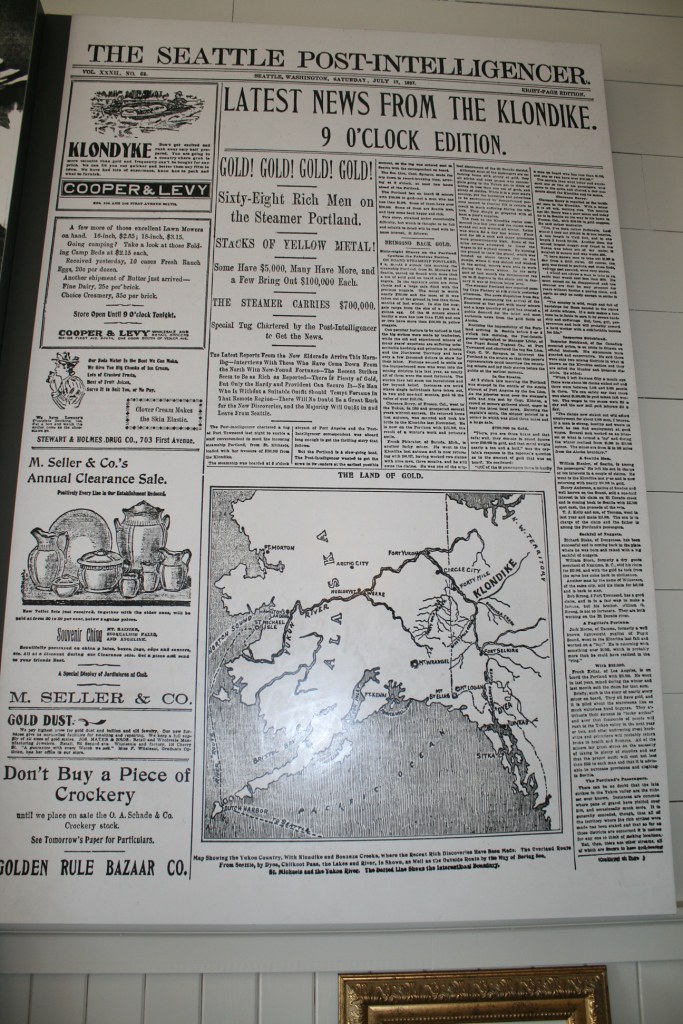The image depicts a detailed zoomed-in photograph of a vintage newspaper page, prominently featuring the header "The Seattle Post-Intelligencer." This newspaper page, showcased as part of an indoor exhibition, appears to be mounted on a white wooden wall, suggesting a possible museum setting. Dominating the center of the image is the newspaper's headline: "Latest news from the Klondike, 9 o'clock edition," followed by the captivating announcement, "Gold, gold, gold, gold. 68 rich men on the steamer Portland. Stacks of yellow metal." The left sidebar of the paper includes advertisements for Cooper and Levy, and M Seller and Company, which promotes items for the kitchen. Just below is an eye-catching slogan: "Don't buy a piece of crockery," associated with the Golden Rule Bazaar. Centrally located at the bottom is a detailed map of Alaska, including the Klondike region, labeled as "the land of gold." Beneath this newspaper page, there appears to be the top edge of a gold-framed picture, further enhancing the historical ambiance of the display. The color scheme of the image includes shades of black, white, gray, gold, and tan, adding to the vintage aesthetic of the scene.